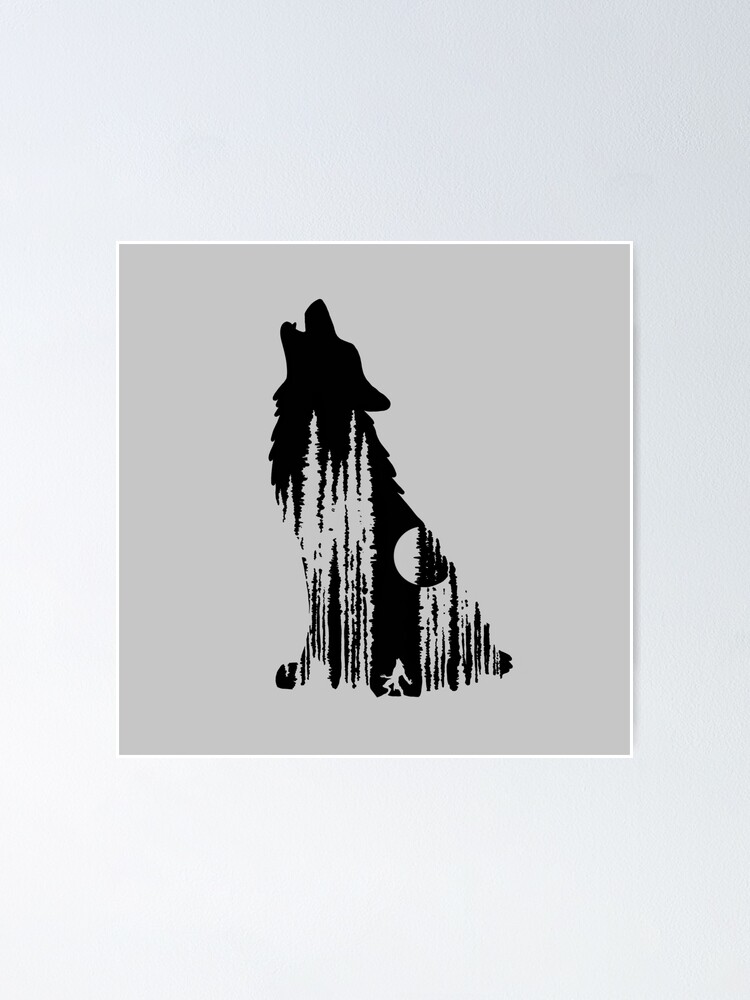The artwork, set against a plain white wall, features a black silhouette of a wolf howling at the moon, placed on a pale gray square background. The style echoes that of a wood block or linoleum block print. Encapsulated within the howling wolf's silhouette are tall, narrow trees, reminiscent of an Alaskan forest, along with an area showcasing part of the moon. Additionally, at the lower section of the wolf's silhouette, there is a small human figure, possibly a hunter holding a spear, adding a layer of intrigue to the scene. This detailed and intricate piece, possibly a silkscreen print, projects a captivating blend of nature and abstract elements, framed by a thin white border and seemingly prepared for display.